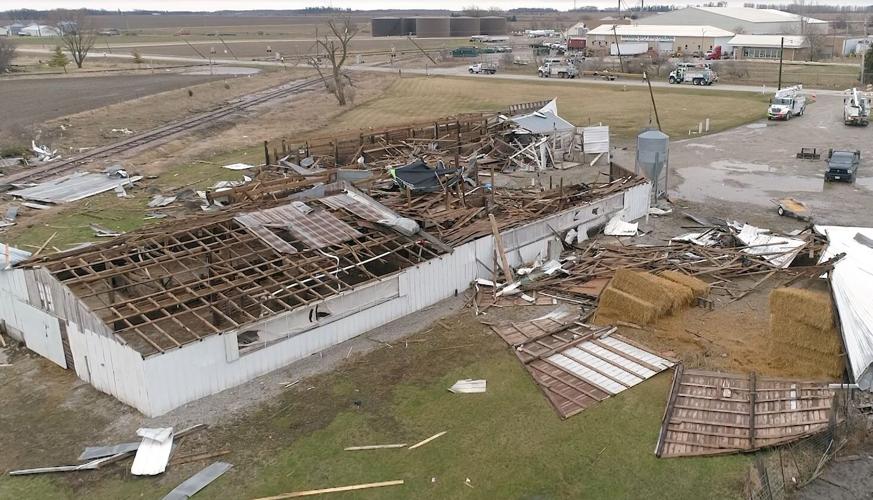This color aerial photograph showcases extensive tornado destruction in a flat, Midwestern farm community, likely in Kansas. The focal point is a large, low, white industrial chicken coop or farm building, approximately a city block long, with its roof completely ripped off and scattered like toothpicks across the ground. Lumber and debris are strewn around the building. Adjacent to this structure, there are bales of hay, possibly once covered in tarps that now lie displaced. A road traverses the upper portion of the image, beyond which stand large unaffected silos and warehouse-like buildings. At least four power company trucks equipped with cherry pickers and possibly a sheriff's vehicle are visible, indicating active recovery efforts. In the lower right, another building lies utterly demolished with its wooden walls flat on the ground as if peeled off. The overall scene epitomizes the aftermath of a devastating tornado in a quintessential American farm setting.